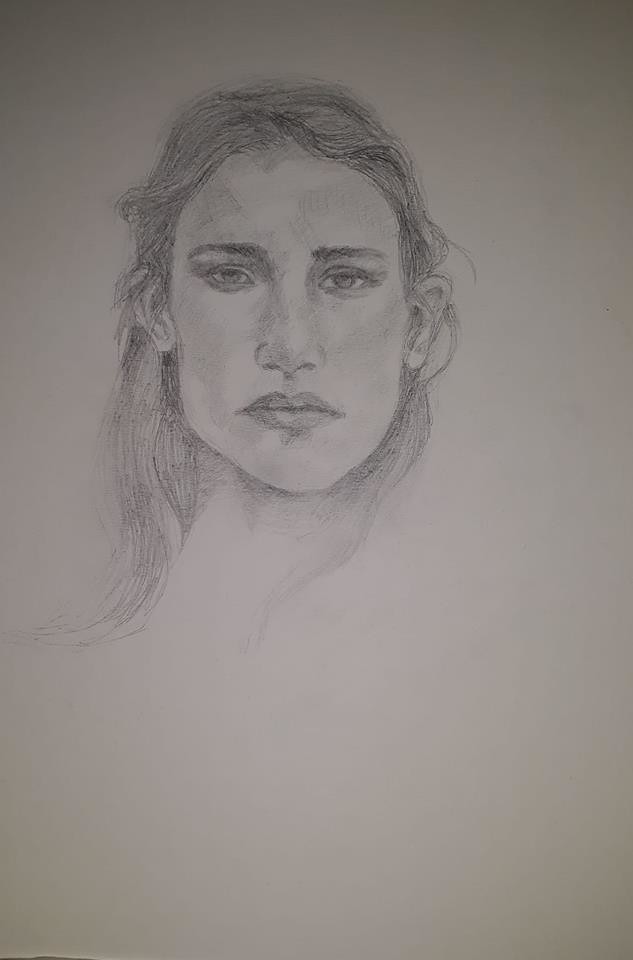The image is a hand-drawn pencil illustration of a woman's face, rendered with meticulous detail and shading. The drawing, done on an off-white or whitish-grey sheet of paper, captures the woman's visage with both her eyes looking straight ahead, exuding a neutral to stern expression. Her full lips are closed, and the nose is well-defined with shading to highlight its contours. She has straight, prominent eyebrows and a slightly strong jawline. Her hair, which is long and reaches past her shoulders, frames her face messily with wisps and curls, tucking behind her ears. Despite the high level of facial detail, the image has a slightly pixelated appearance and darker edges, suggesting it is a photograph taken under low light or with a low-quality camera. Only her neck is partially visible, with no other parts of her body shown.